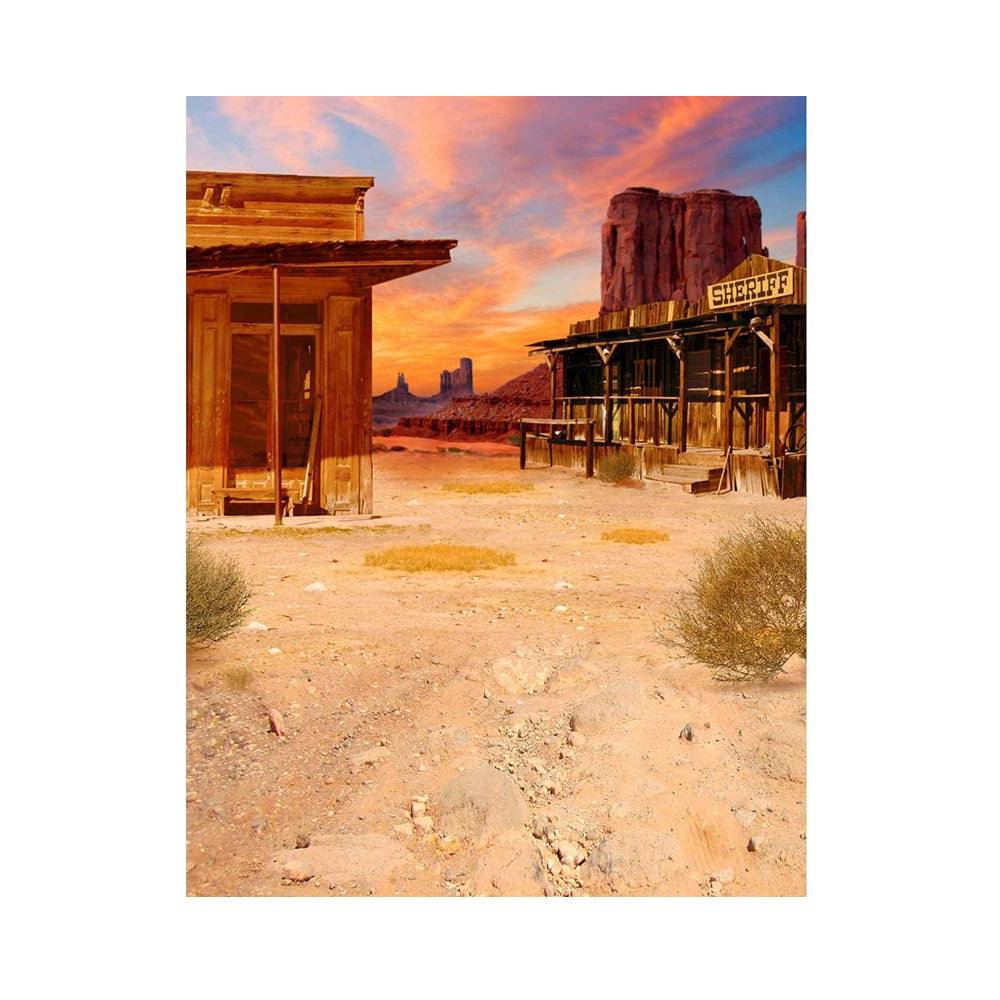A digital portrait mode image depicts an evocative scene from the Wild West at sunset. The bright blue sky transitions seamlessly into a stunning array of reds, oranges, and yellows as the sun sets behind a range of purple and dark pink mountain formations that jut sharply into the sky. These rugged peaks form a dramatic backdrop for the scene.

In the foreground, the image captures the essence of an old, possibly deserted western town. Two wooden buildings dominate the scene: to the left is a nondescript building with a bench outside, its purpose unknown, while to the right stands the Sheriff's office, clearly labeled and equipped with a doorstep and a small porch. This office features a wooden structure to tie up horses, enhancing the historic atmosphere.

The streets and surroundings are composed of dirt and sand, with hues of white, yellow, and orangish-brown that blend with patches of yellow-brown grass and sparse green bushes. Tumbleweeds lie scattered across the barren ground, emphasizing the deserted feel of the town. The subtle clouds in the sky contrast gently with the vibrant sunset, adding to the serene yet stark beauty of this wild western landscape.